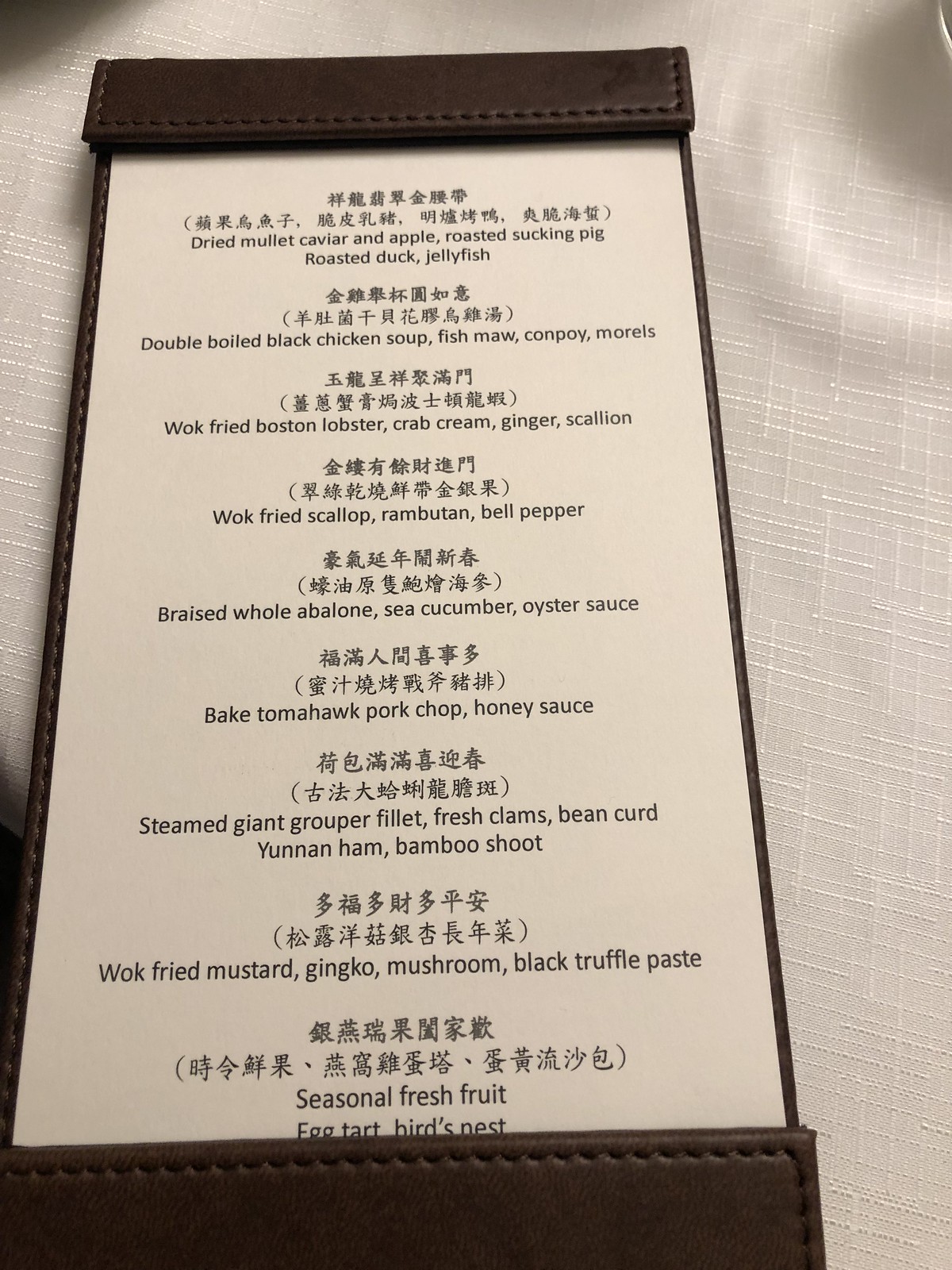This is a color photograph featuring a Chinese menu displayed on a white, textured cloth background. The top and bottom sections of the menu are adorned in brown leather, lending it an elegant and sophisticated appearance. The menu showcases a variety of Chinese dishes, each with Chinese characters accompanied by English translations for better understanding.

Starting from the top, the dishes include:

1. Dried mullet caviar and apple
2. Roasted suckling pig
3. Roasted duck
4. Jellyfish
5. Double boiled black chicken soup
6. Fish maw
7. Conpoy (dried scallops)
8. Morels
9. Wok-fried Boston lobster, complemented by crab cream, ginger, and scallion
10. Wok-fried scallop with rambutan and bell pepper
11. Braised whole abalone
12. Sea cucumber in oyster sauce
13. Baked tomahawk pork chop with honey sauce
14. Steamed giant grouper fillet with fresh clams, bean curd, Yunnan ham, and bamboo shoot
15. Wok-fried mustard with ginkgo and mushroom in black truffle paste
16. Seasonal fresh fruit
17. Egg tart
18. Bird's nest

Each listed item reflects the rich and diverse culinary traditions of Chinese cuisine, offering a blend of traditional flavors and contemporary presentations.